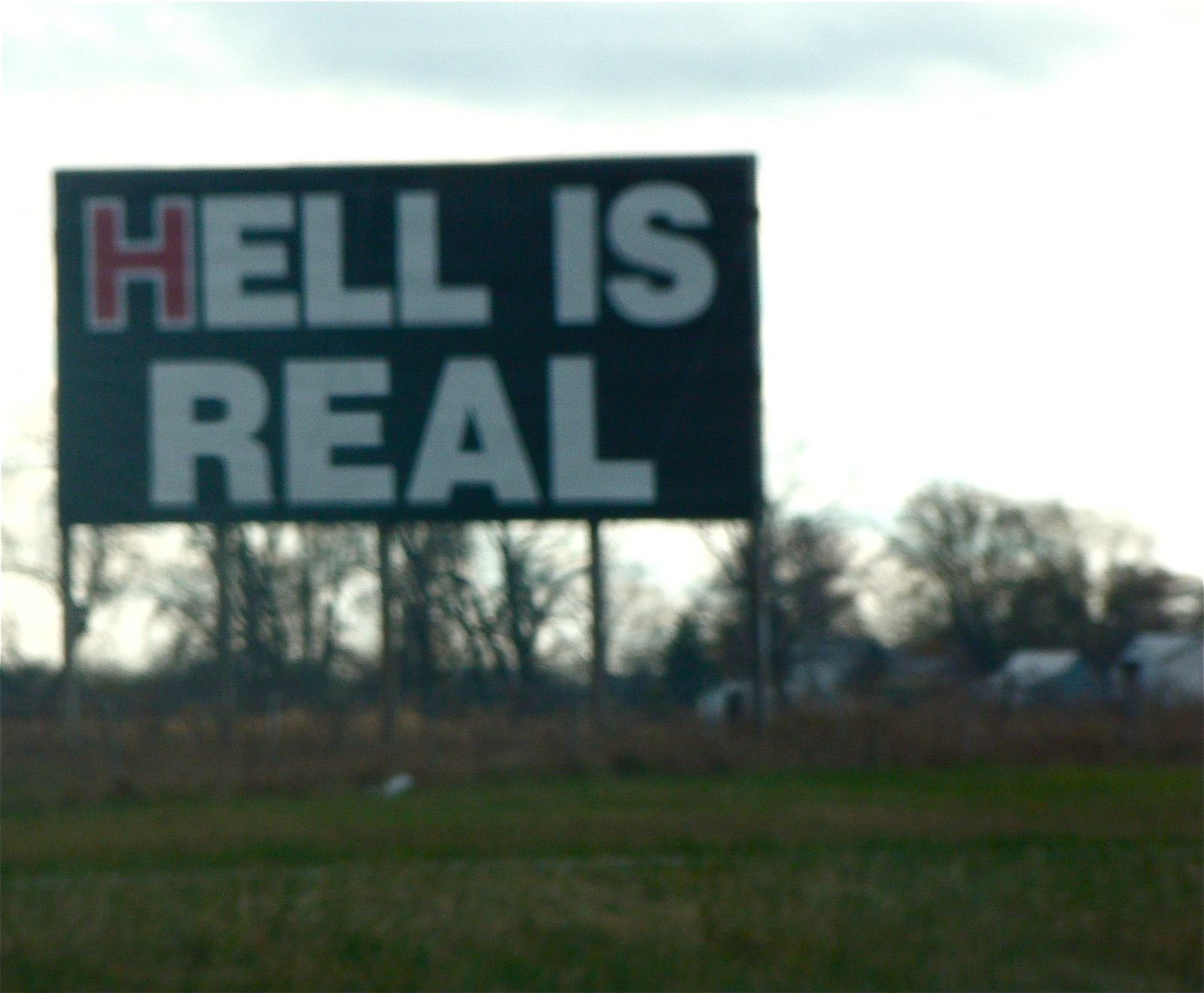This is a blurry, low-light color photograph taken at dusk or with a filter, leading to poor lighting. The image prominently features a large rectangular billboard centered slightly left. The billboard has a black or very dark blue background and is supported by multiple dark metal posts standing in a grassy field. Written on the billboard in all caps are the words "Hell is real," with the "H" in Hell outlined in white and filled with red, and the remaining letters in white. Above the billboard, the sky is almost entirely overcast with heavy clouds, except for a small patch of light blue peeking through at the top. Behind the billboard, lining the background, are silhouettes of trees, and to the far right, partially obscured by the vegetation, stand a few white buildings.